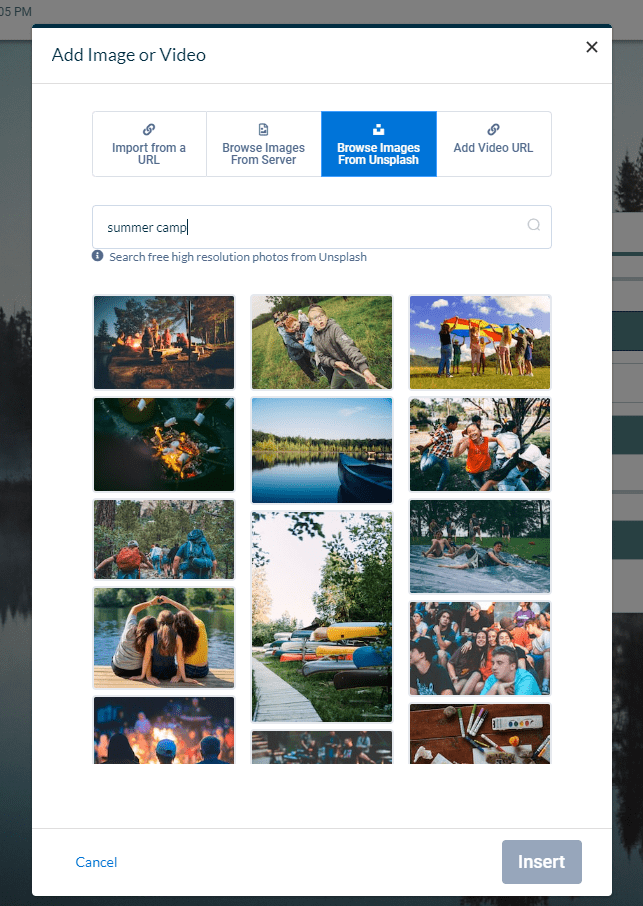In this image, a person appears to be using a device, likely a phone or tablet, to transfer or manage pictures through a specific application. At the top of the screen, a white rectangle is superimposed over another open program, indicating a multi-tasking interface. The top part of the rectangle features an instruction to "Add Image or Video," accompanied by four distinctive icons. The first icon reads "Import from a URL," the second instructs to "Browse Images from a Server," the third, highlighted in blue with white text, says "Browse Images from Unsplash," and the fourth icon offers "Add Video URL."

Below these options, there's a rectangular banner designed to function as a search bar with the placeholder text "Summer Camp." Underneath this, it elaborates with "Search free high resolution from Unsplash," suggesting that this is an application or interface related to Unsplash, a popular source for free high-resolution images.

The main section of the screen is divided into three columns displaying various camp-related photographs. These images include scenes of friends sitting on a dock, canoes stacked on grassy terrain beside a water body, a group picture of boys and girls smiling, friends playing and splashing in water, and friends holding up what looks like a tent or parachute. Overall, the images evoke a lively and nostalgic atmosphere of summer camp activities.